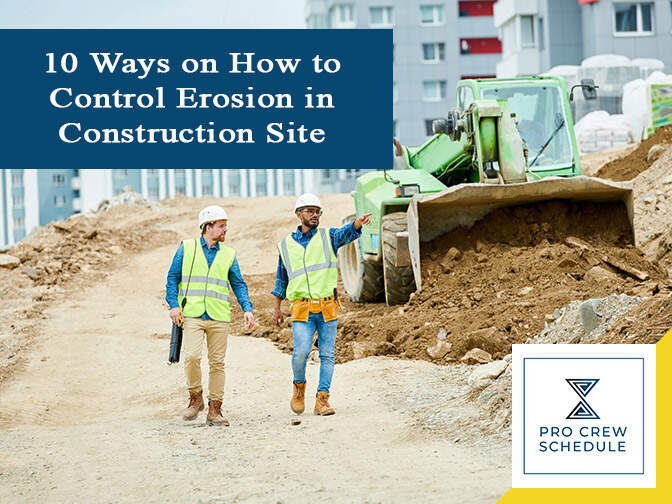The front page of an ad or informational booklet features a detailed scene of a construction site. The foreground shows two men walking side by side down a dirt path, both sporting white hard hats and neon yellow reflective vests over blue long-sleeved shirts. One wears denim pants while the other dons khaki pants, both completing their outfits with brown safety boots. One of the men, likely in charge, is actively pointing, presumably giving directions. To their right, a green excavator filled with dirt is prominently engaged in its task. The background reveals some blue-tinted, concrete apartment buildings. At the top left, a blue rectangle with white text reads, "10 ways on how to control erosion in a construction site." In the bottom right corner, a yellow-bordered white box states "Pro Crew Schedule" alongside a symbol, indicating the company or consultancy providing the information.